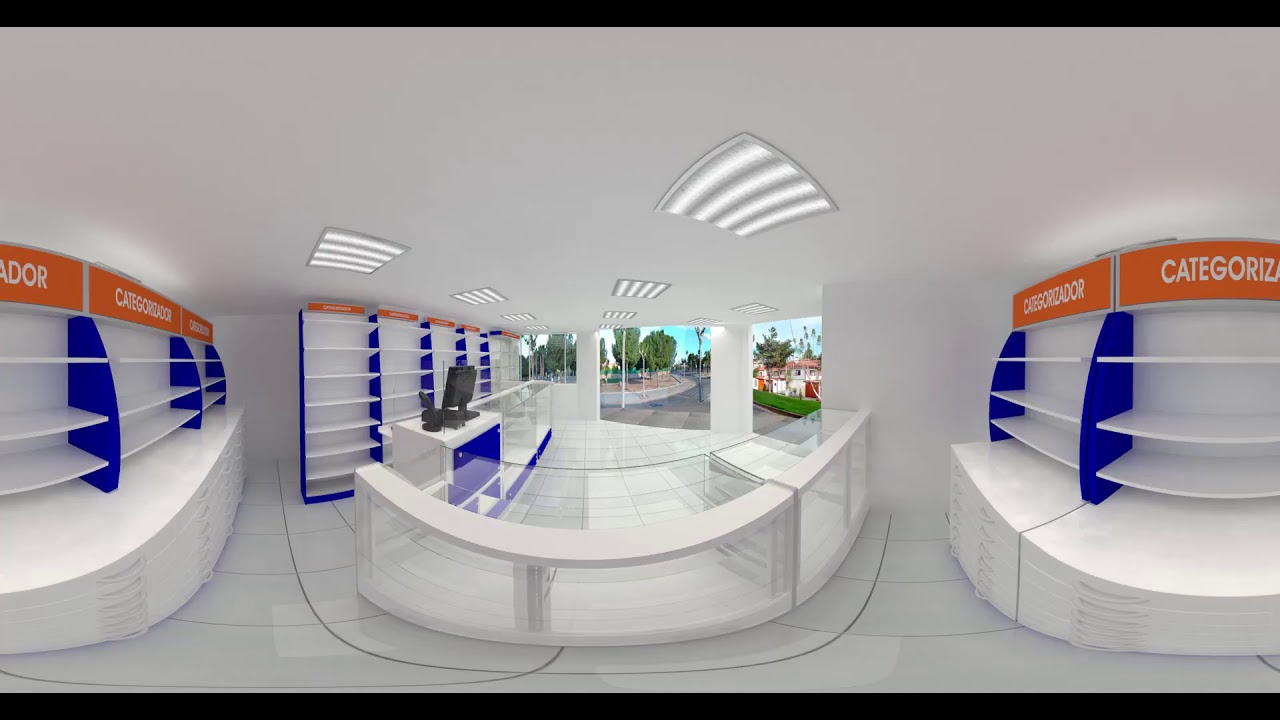The image depicts the interior of a large, mostly white building, possibly an unused store or newly constructed facility. The central focus is the main entryway, which leads to a room with glass cases and white countertops, likely meant for displaying products like jewelry or electronics. Behind these counters are additional areas for storage, featuring extensive white shelving with blue dividers. Prominent orange signs with white lettering, including one that reads "Categorizador," are visible on the shelving. A small desk with a point-of-sale system, a computer, and a scanner is also present, indicating operational capabilities. The building has a white ceiling adorned with square recessed lights and large windows that offer a view of trees, a road, grass, and some distant buildings. All these elements are placed on a white tile floor, and no people are visible in the scene, giving it an empty, pristine appearance.